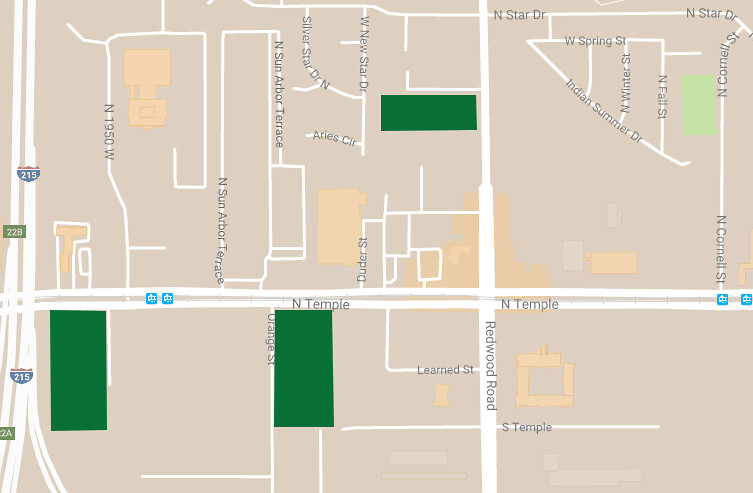This is a detailed screenshot of a street map displayed on a computer, featuring a beige background for ease of viewing. The map highlights various buildings depicted in light brown, along with several smaller outbuildings that appear in a slightly lighter shade of beige. Positioned on the left side of the map are three large rectangles. 

A major highway runs vertically down the left side of the map, curving towards the right at the bottom. This highway is marked with a blue and red shield bearing the number "215" prominently in white. Additionally, there are two rectangles indicating the exit numbers "22B" and "22A" for this highway.

Centrally located, a cross-street labeled "North Temple" runs horizontally across the map. Slightly to the right of the map's center, a significant vertical road labeled "Redwood Road" can be seen. Adjacent to the left side of the highway, there are two small blue squares each featuring a white symbol at their center, marking specific points of interest or facilities. This descriptive map provides a comprehensive view of the area's layout, key roads, and essential landmarks.